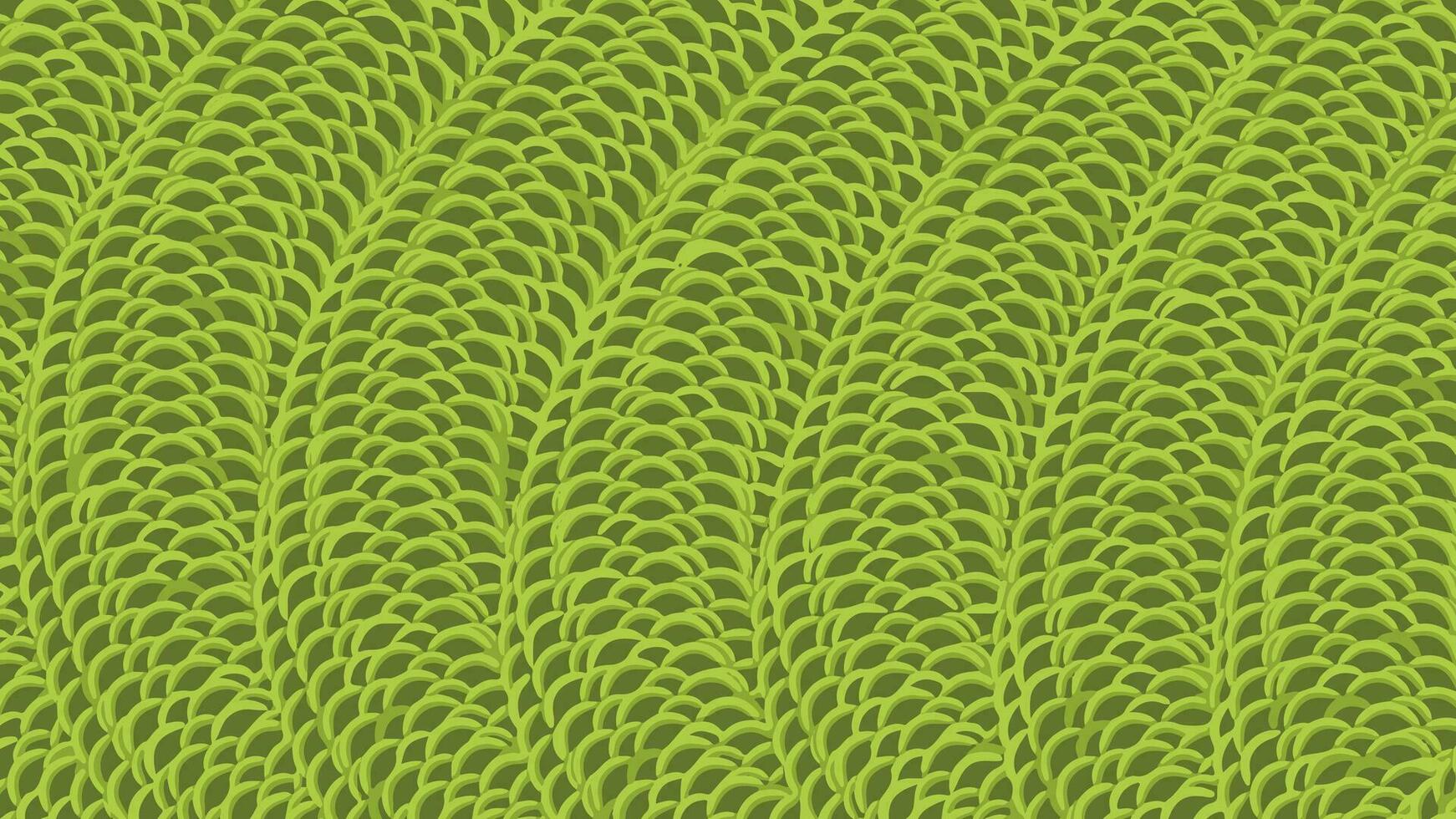The image is a detailed color illustration with a repetitive pattern reminiscent of snakeskin or woven rope. It features seven neatly aligned coils, resembling a water hose wound side by side, all set against a solid dark olive green background. The coils vary slightly in shape and are intricately detailed with what appear to be scales or ridges. The scales are highlighted with neon green on their outer edges, creating a striking contrast with the darker green beneath. The overall pattern is continuous and tightly packed, running seamlessly from left to right and top to bottom in a landscape orientation, evoking the appearance of a meticulously crafted textile art piece. The vivid green hues give the coils a somewhat slimy, bright, and almost luminescent quality, enhancing the intricate details of the pattern that covers the entire image.